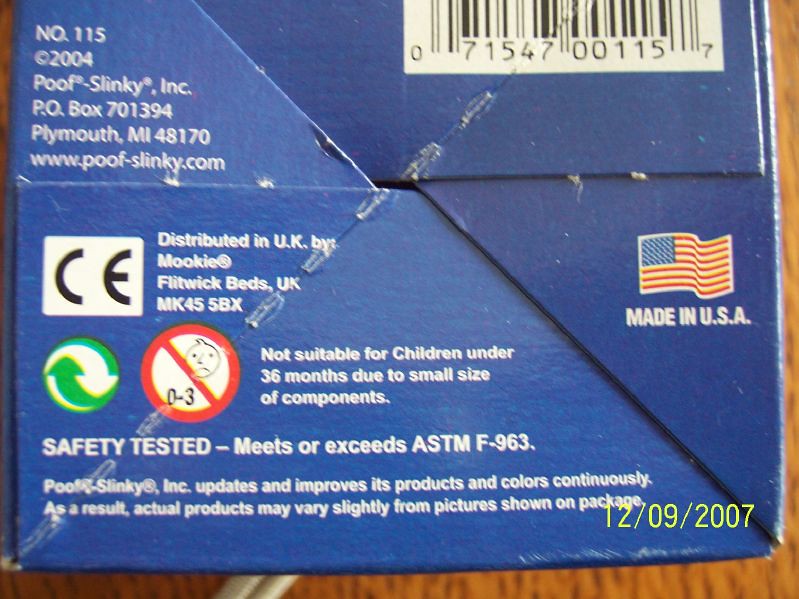The photograph captures the bottom of a blue box set against a wood grain background. In the upper right corner, a barcode is clearly visible. Below the barcode, an American flag is prominently displayed with the text "Made in USA" in white beneath it. In the upper left corner, the notation "NO115" appears next to a copyright mark indicating the year 2004, followed by "POOF Slinky Inc." Additional details include a P.O. Box address in Plymouth, MI 48170, and a website link to www.poof-slinky.com. Various icons are also present, including a CE mark, a green recycling symbol, and a crossed-out icon signifying that the product is not suitable for children under 36 months due to small parts. An annotation mentions that the product meets or exceeds safety standards, and there's a time stamp in the lower right corner dated 12-09-2007.